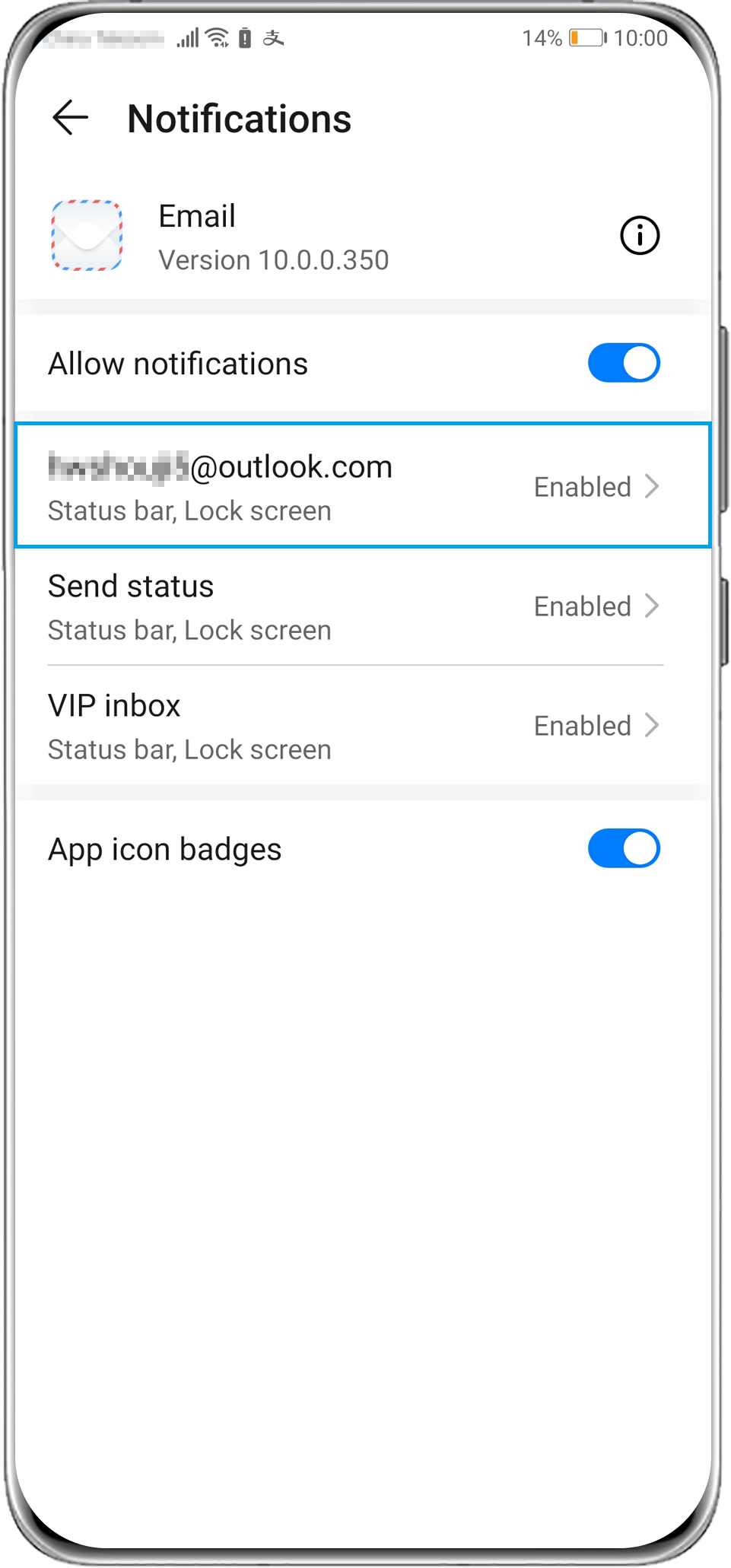The screenshot displays a smartphone interface at 10 o’clock, indicated by a status bar showing a 14% battery level. The screen contains various settings under a section labeled "Notifications" for an email application, version 10.0.0.350. At the top, there's a left-pointing arrow, allowing navigation back to the previous screen. Below it is an oval icon with a lowercase "i" inside, representing information, and next to it is the option "Allow notifications," which is enabled with a blue toggle bar.

Beneath this section, a blue-outlined box highlights an email address that is partially blurred for privacy, identifiable only as belonging to the "@outlook.com" domain. Several options follow, indicating the status for various notification settings:

- **Status Bar** and **Lock Screen**: Both are enabled.
- **Send Status**: Enabled on the status bar and lock screen.
- **VIP Inbox**: Enabled on the status bar and lock screen.
- **App Icon Badges**: Enabled with a blue toggle bar.

The rest of the screen displays blank space extending to the bottom, suggesting no additional settings or information are present.